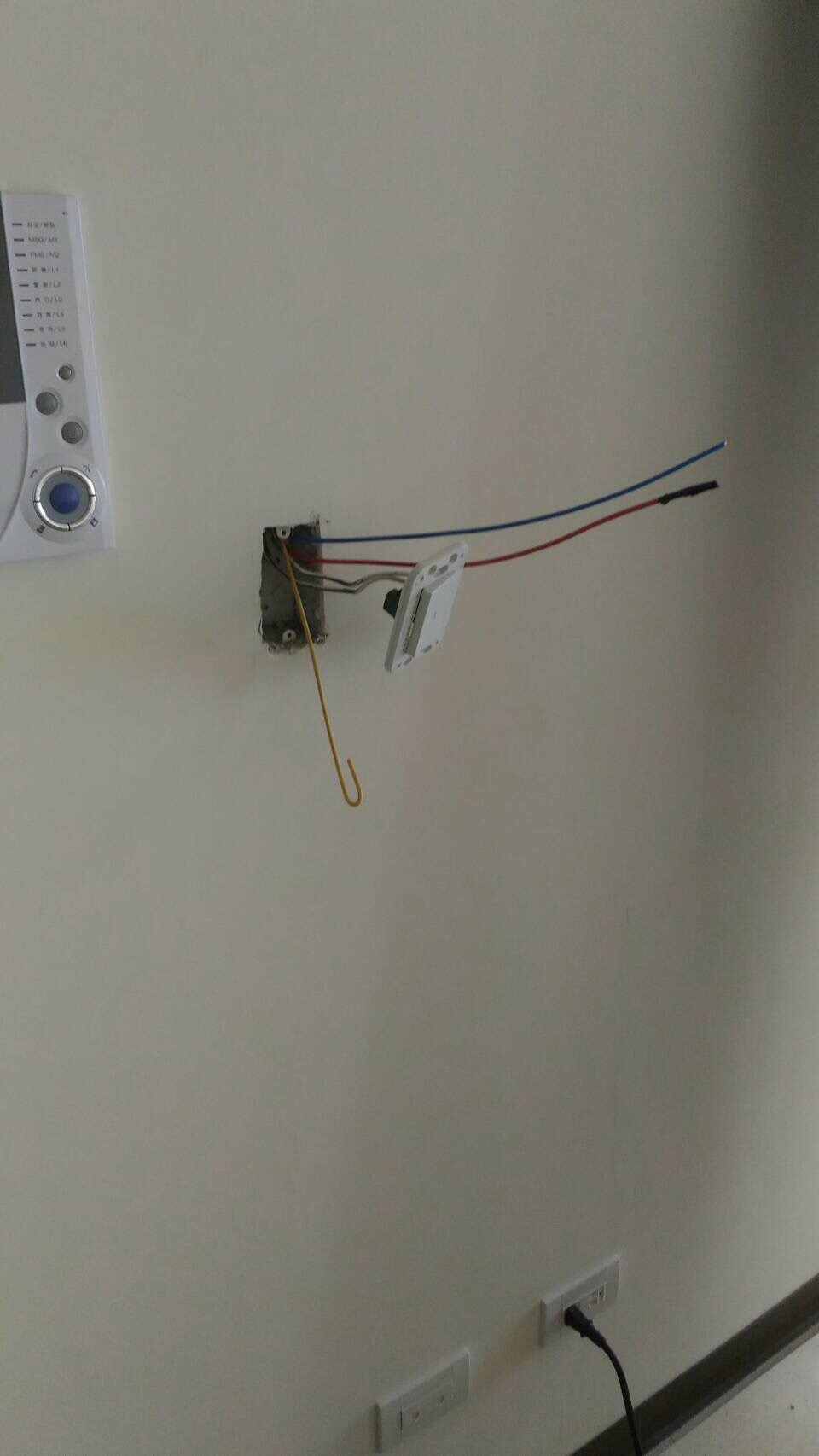The image depicts a white rectangular wall with various electrical fixtures. At the bottom, the wall is bordered by a black trimming. Two electrical outlets are located side by side at the base of the wall, with one outlet currently occupied by a black plug.

Moving upwards, there is an uncovered outlet, revealing the inner wiring and structure. Through a square or rectangular cutout in the wall, a blue wire and a red wire with electrical tape at the end protrude. Additionally, a metal plate, intended for securing the outlet, is visible, along with a hook emerging from the electrical box.

Towards the upper left section of the wall, part of a thermostat is visible, showing only its right side with a few gray buttons. The overall color of the wall is white.